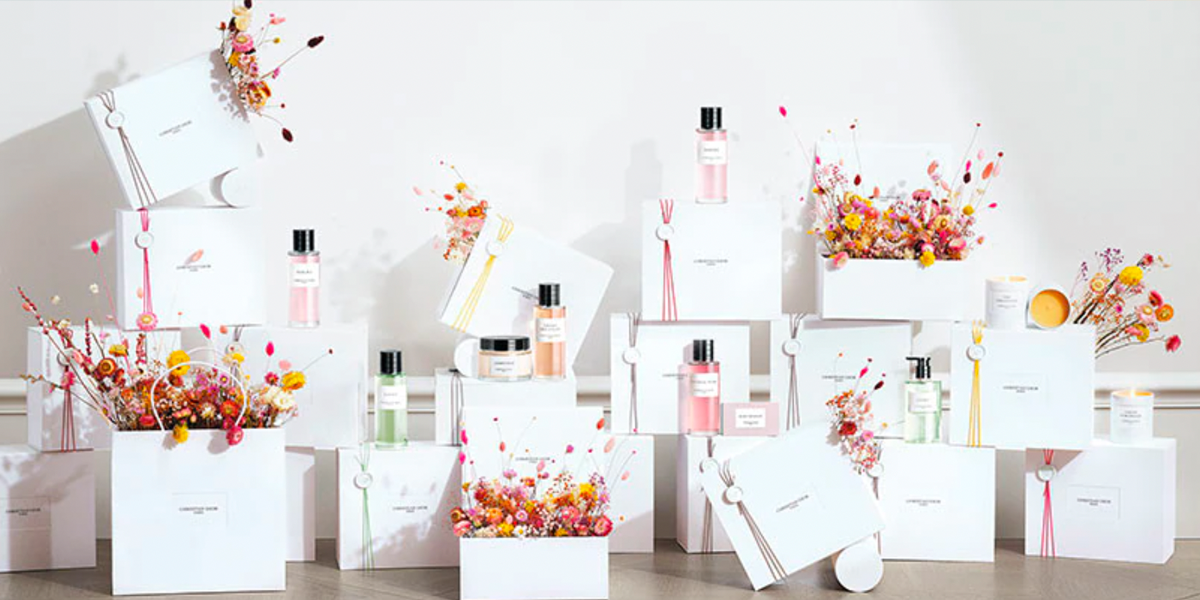The image depicts a detailed display of personal care giveaways, including a collection of clear glass jars with shiny black tops, filled with various soaps, creams, and possibly fragrances. These products, appearing in hues of pink, light pink, orange, and light green, are meticulously arranged atop a series of white gift boxes and bags, which a total of around 20 to 22, all similar in size and shape. Adding a touch of color and vibrancy to the scene, red and orange artificial flowers, some with orange and red stems, emerge from a few boxes and bags. The arrangement is set against a clean white wall with a baseboard, creating a striking contrast. The variety of bottles includes those that appear to contain gels or sprays, centrally positioned, alongside additional items like jars of creams and potentially candles, making it an eye-catching and cohesive display of diverse personal care products.